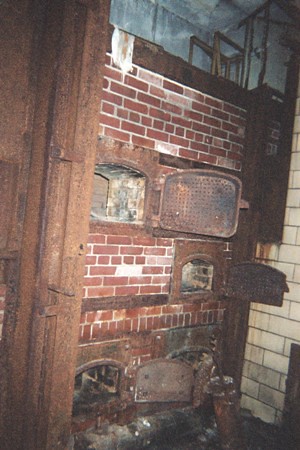This image is a color photograph depicting an abandoned building, possibly an old restaurant or industrial facility. The central focus is a red brick wall featuring three rusted, old-style oven doors; all of which are open. The top door is partially sealed with brown wood, while the bottom door is surrounded by dirt. The brick wall also contains white bricks arranged in a slab pattern, which are heavily stained and rust-marked, suggesting long-term neglect. To the left, a brown door frame and a closed brown door are visible, and to the right, a dirty white brick wall. The photograph is shot in portrait mode, emphasizing the aged and decrepit condition of the structure, devoid of any people, animals, or modern vehicles.